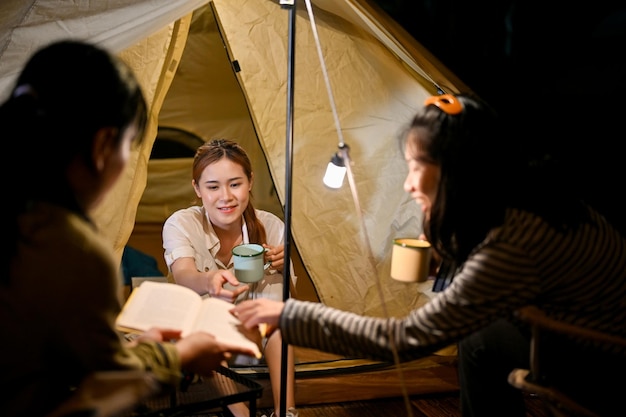In this captivating nighttime outdoor photograph, three Asian women are seated in front of a triangular tent, enveloped in the gentle glow from a light attached to the tent pole. Dominating the scene, the woman in the middle, with long brownish hair, is dressed in a white t-shirt and shorts. She holds a light green metal mug in one hand and is smiling as she points towards a book. To her left, partially obscured in the bottom-left corner of the image, another woman has her back turned, also holding an open book. On the right, a third woman with black hair, adorned with an orange headband, wears a long-sleeved gray and black striped shirt. She holds an orange mug similar in style to the green one and is also pointing towards the book. The tent, a dark tan color with a white tarp roof, provides a cozy backdrop to this serene and intimate moment, captured in the stillness of night.